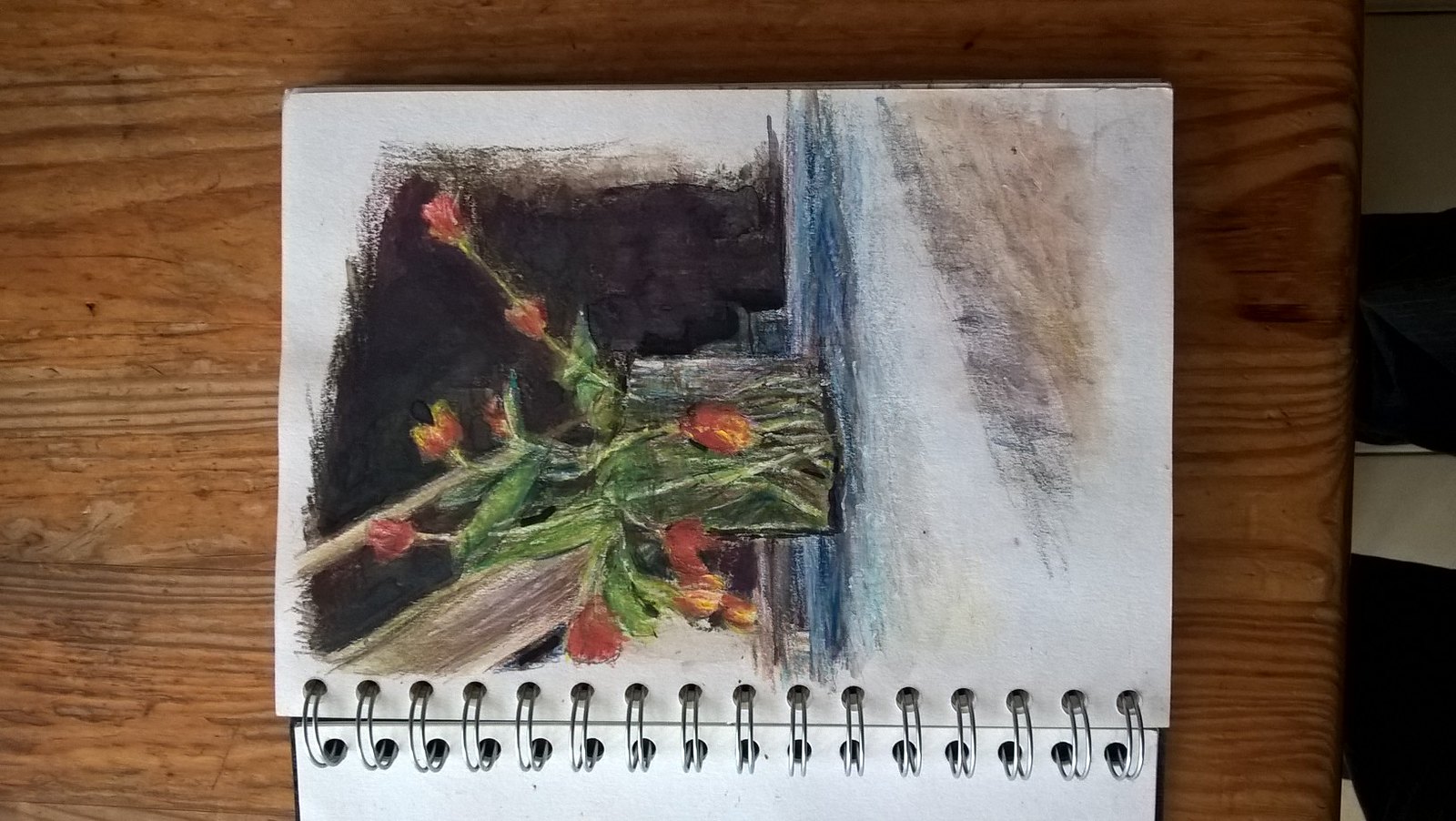This image shows a top-down view of a spiral-bound notebook laid horizontally on a wooden table, with the spiral part facing downwards. The notebook's top page features a drawing of a vase with red and orange flowers that resemble tulips, approximately eight to ten in number, some of which drape over the edge of the vase. The vase sits on a surface drawn in varying shades of blue and black, transitioning to a lighter gray outside the base area. In the background of the drawing, there is a window depicted in black with brown lines on its left side and some angled, wood-like tan shapes extending towards the top left of the image. The scene is illuminated more brightly on the left side, casting shadows to the right. Additionally, to the right of the notebook on the table, there are black and white striped fabrics.